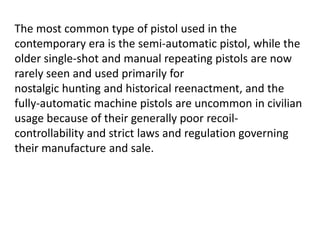In the image, there is a text write-up presented on a small, thumbnail-like white background with clear black text. The text reads: "The most common type of pistol used in the contemporary era is the semi-automatic pistol. While older single-shot and manual-repeating pistols are now rarely seen and are primarily used for nostalgic hunting and historical reenactment, fully automatic machine pistols are uncommon in civilian usage due to their generally poor recoil controllability and strict laws and regulations governing their manufacture and sales." The left side of the text is indented, while the right side is not.